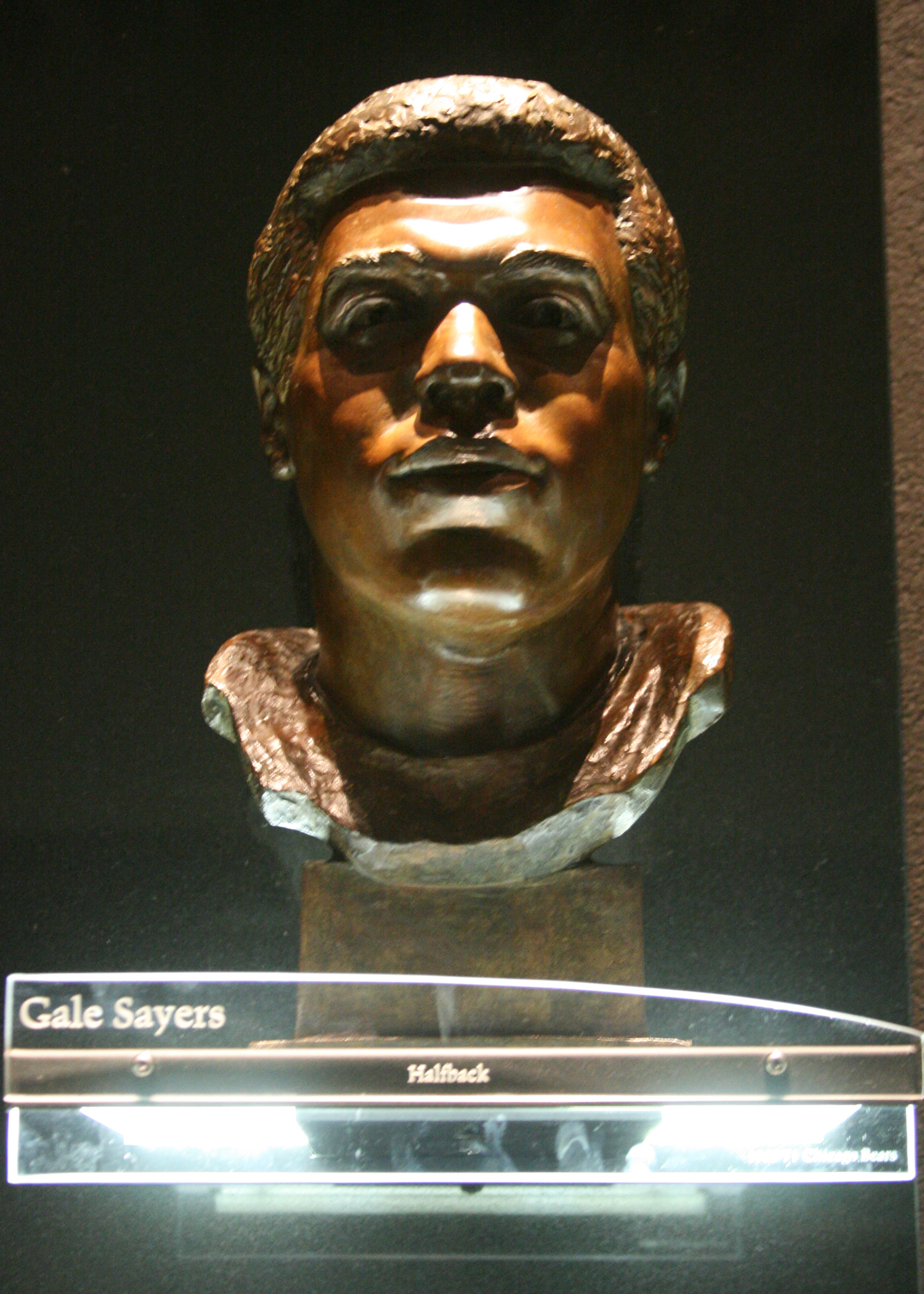This image features a detailed bronze sculpture of Gale Sayers, a former NFL half-back renowned for his time with the Kansas Comet. The bust is meticulously molded, capturing the essence of Sayers' head, and is displayed in a football hall of fame. The sculpture exudes a golden and brown hue, achieved through its bronze, copper-ish material. It is mounted on a translucent pedestal that bears his name and position, "Gale Sayers" and "Half-Back." The display is highlighted by lighting from both above and below, casting intriguing shadows and vertical stripes, with a subtle brown backdrop enhancing the overall presentation.